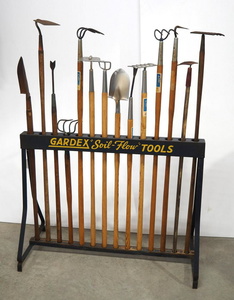The image showcases a black metal rack against a white wall, positioned on a gray floor, holding an assortment of roughly 12 garden tools. The tools include a spade, multiple rakes, shovels, hoes, a weeding tool, a small pitchfork, a cutter, and other varied gardening implements. Each tool is inserted into corresponding holes at the top and base of the stand, ensuring an organized and upright arrangement. Prominently displayed on the upper front of the rack, in golden yellow font, is the label "Gardex Soil Flow Tools." A noticeable shadow appears to the left, cast from an object outside the image frame. The rack's design includes dual legs for stability and serves as a convenient and tidy storage solution for gardening tools.